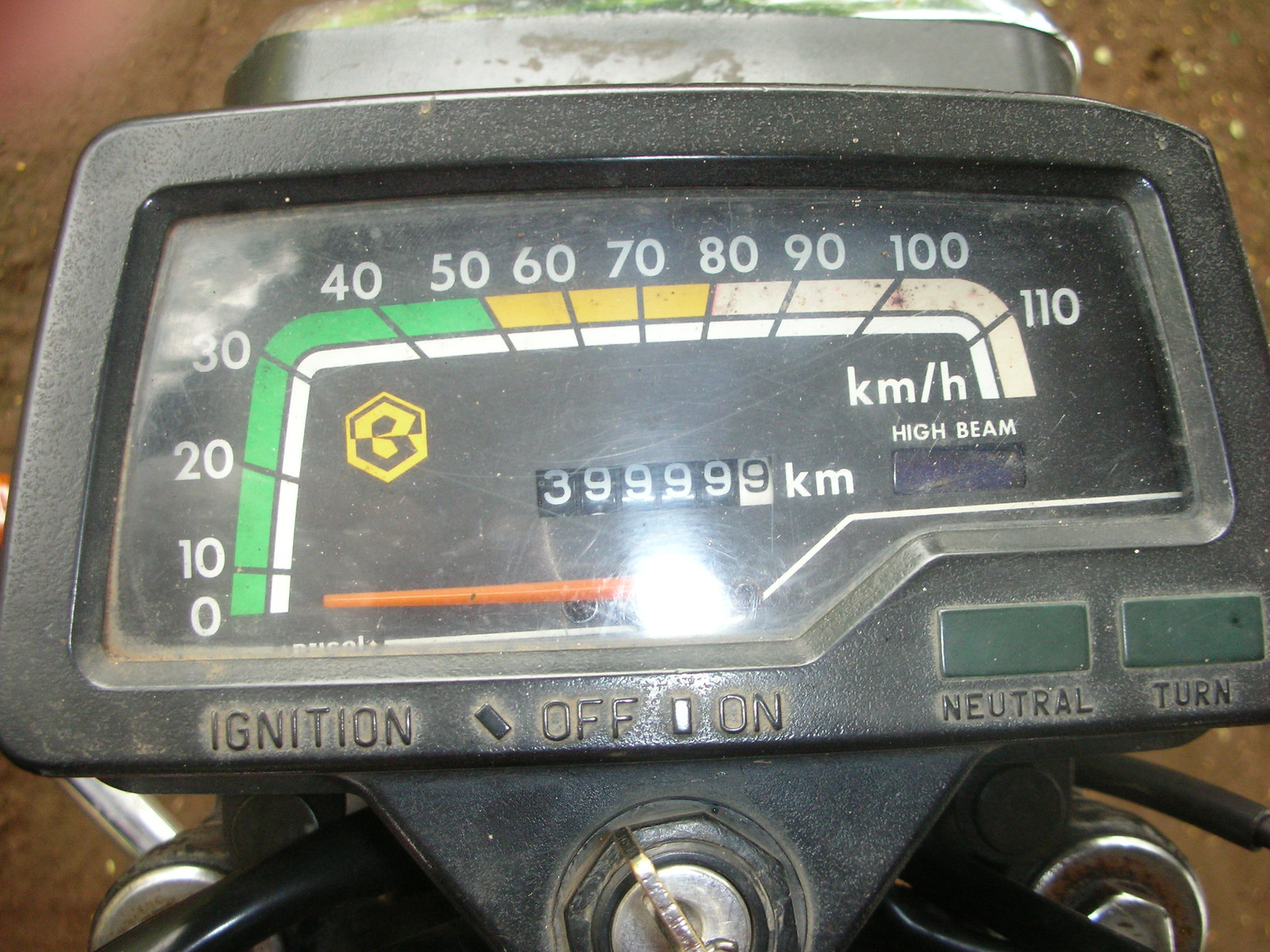The color photograph, captured in landscape orientation, provides a bird's eye view directly down at the speedometer and odometer of a two-wheeled vehicle, likely a scooter or motorbike. The frame encasing the instruments is made of black plastic, heavily soiled with grime and dried brown mud, emphasizing the vehicle's well-used condition.

Along the bottom edge of the frame, various text labels are stamped and slightly raised, adding a tactile quality to their appearance. From left to right, the labels read "IGNITION," followed by "OFF," "ON," "NEUTRAL," and "TURN." Each label is surrounded by patches of dried mud, highlighting their raised surfaces.

The speedometer, situated prominently in the center, displays a zero reading, indicated by an orange needle pointing to the left. Its shape is nearly square, with the numbering beginning at zero in the bottom left corner. The scale ascends to 30, then curves horizontally, stretching to 100, and finally bending downwards to 110.

Adjacent to the speedometer is the odometer, showing a reading of 39,999 kilometers. The last digit, a nine on a white background, contrasts against the black background with white numbers on the other digits.

Visible just below the speedometer's outer casing is a key positioned at a 10 o'clock angle. At the bottom of the image, emerging from the plastic housing, are the beginnings of two black handlebars, one on either side, further confirming the two-wheeled nature of the vehicle.